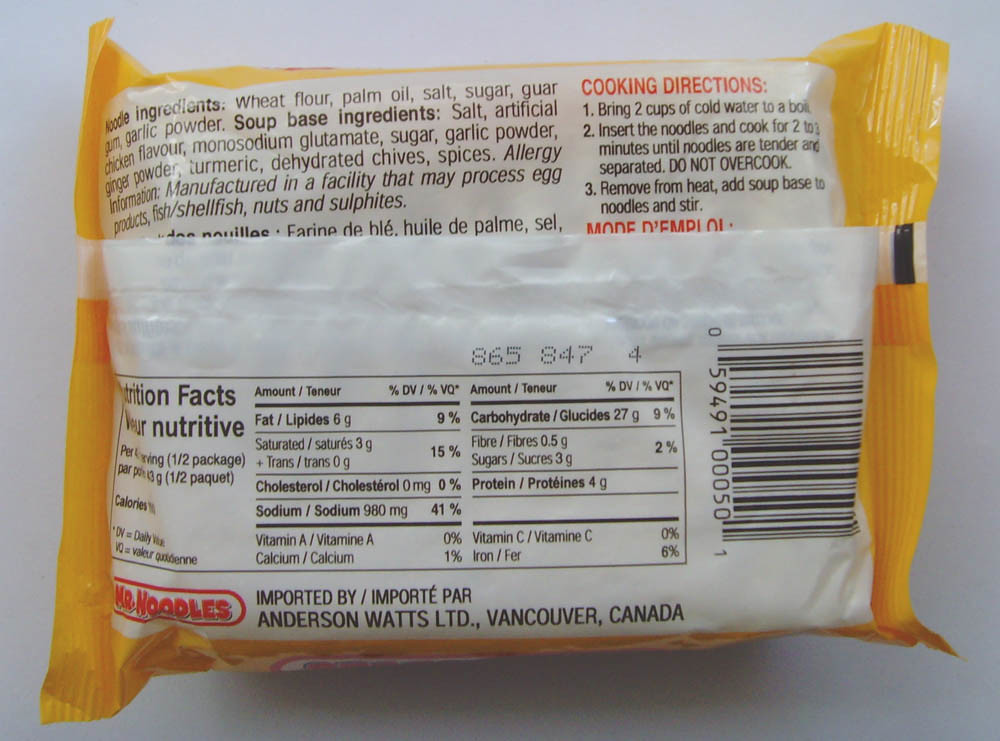This image depicts the back of a noodle packet, providing detailed information about its ingredients, allergy warnings, and cooking instructions. The listed ingredients for the noodles include wheat flour, palm oil, salt, sugar, guar gum, and garlic powder. The soup base ingredients are detailed as salt, artificial chicken flavor, monosodium glutamate, sugar, garlic powder, ginger powder, turmeric, dehydrated chives, and various spices.

Additionally, the packaging contains allergy information, noting that the product is manufactured in a facility that may process egg products, fish, shellfish, nuts, and sulfites. Accompanying this, there is a picture illustrating the cooking directions: bring two cups of cold water to a boil, add the noodles, and cook for two to three minutes until the noodles are tender and separated, with a caution not to overcook.